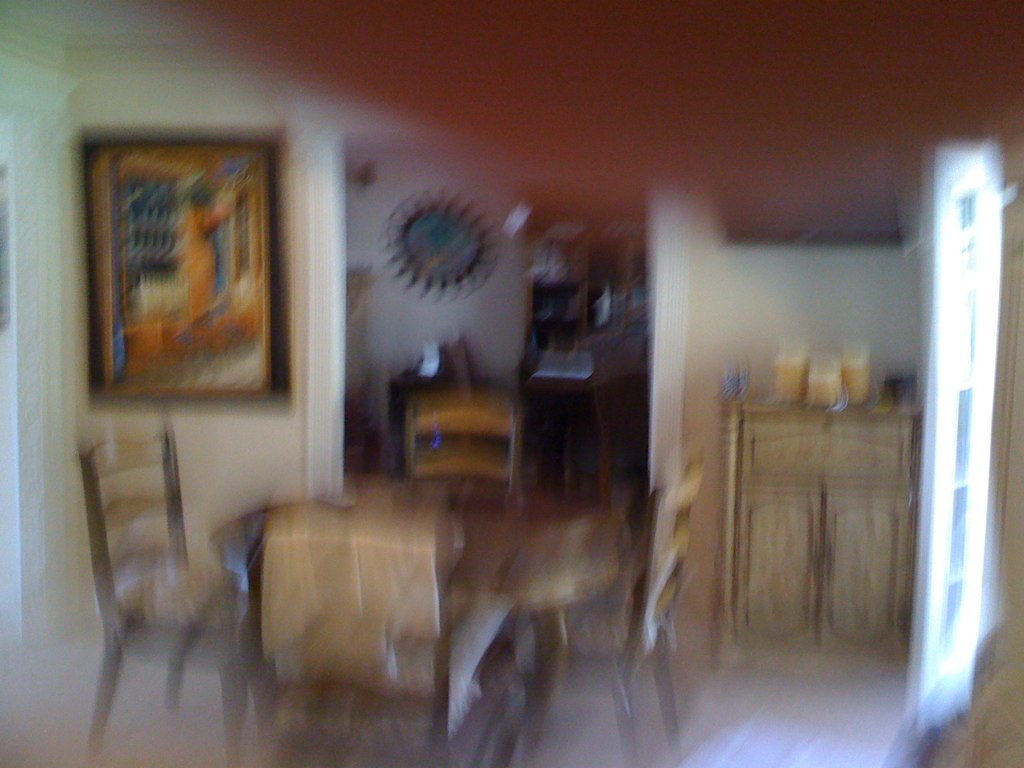Captured in the cozy setting of a living or dining room, this image showcases a charming wooden table accompanied by four matching chairs partially pulled out. The walls, painted a pristine white, serve as a backdrop for various colorful paintings. A quaint mini cabinet, topped with three vibrant yellow candles, adds a touch of warmth and cheer to the scene. To the right, a door subtly integrates into the inviting atmosphere, suggesting a passage to other parts of the home.